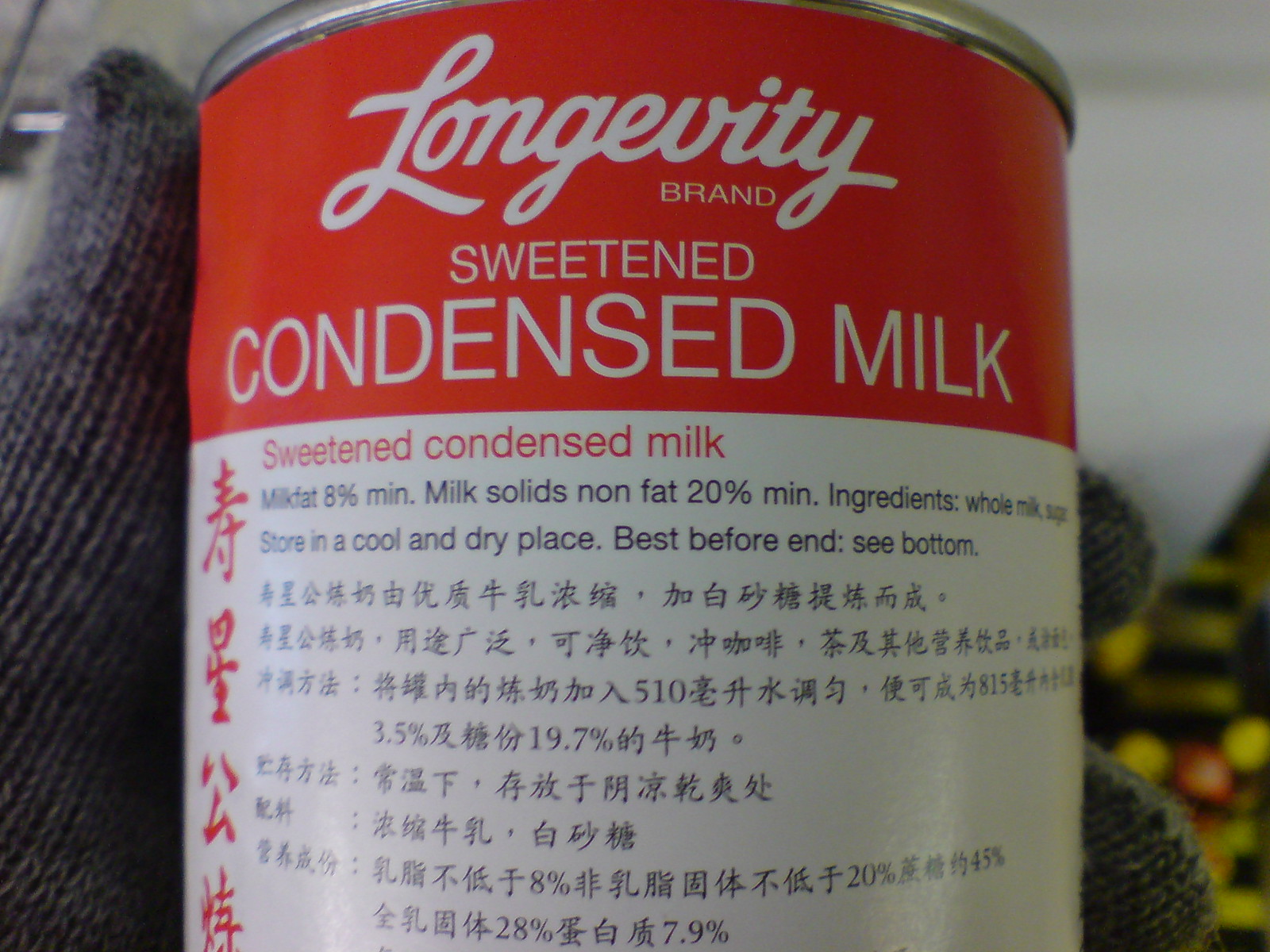In this rectangular close-up photograph, a canned product with a silver top is displayed prominently. The side or back label of the can is divided into two distinct sections: the top third is a vibrant red with white cursive text, and the bottom two-thirds is white with a mix of black and red print. 

The top part of the red section features "Longevity Brand" in elegant cursive white lettering. Directly below that, in a more standard print, it states "Sweetened Condensed Milk." Moving to the white section of the label, the text reads "Sweetened Condensed Milk" again, followed by details regarding its contents: "Milk Fat 8% Min" and "Milk Solids Non-Fat 20% Minimum." 

The ingredients listed are "whole milk, sugar." Further instructions note, "store in a cool and dry place," and "best before end, see bottom." Below these instructions, additional text appears in what seems to be a Chinese script, although the exact language is not certain from the image.